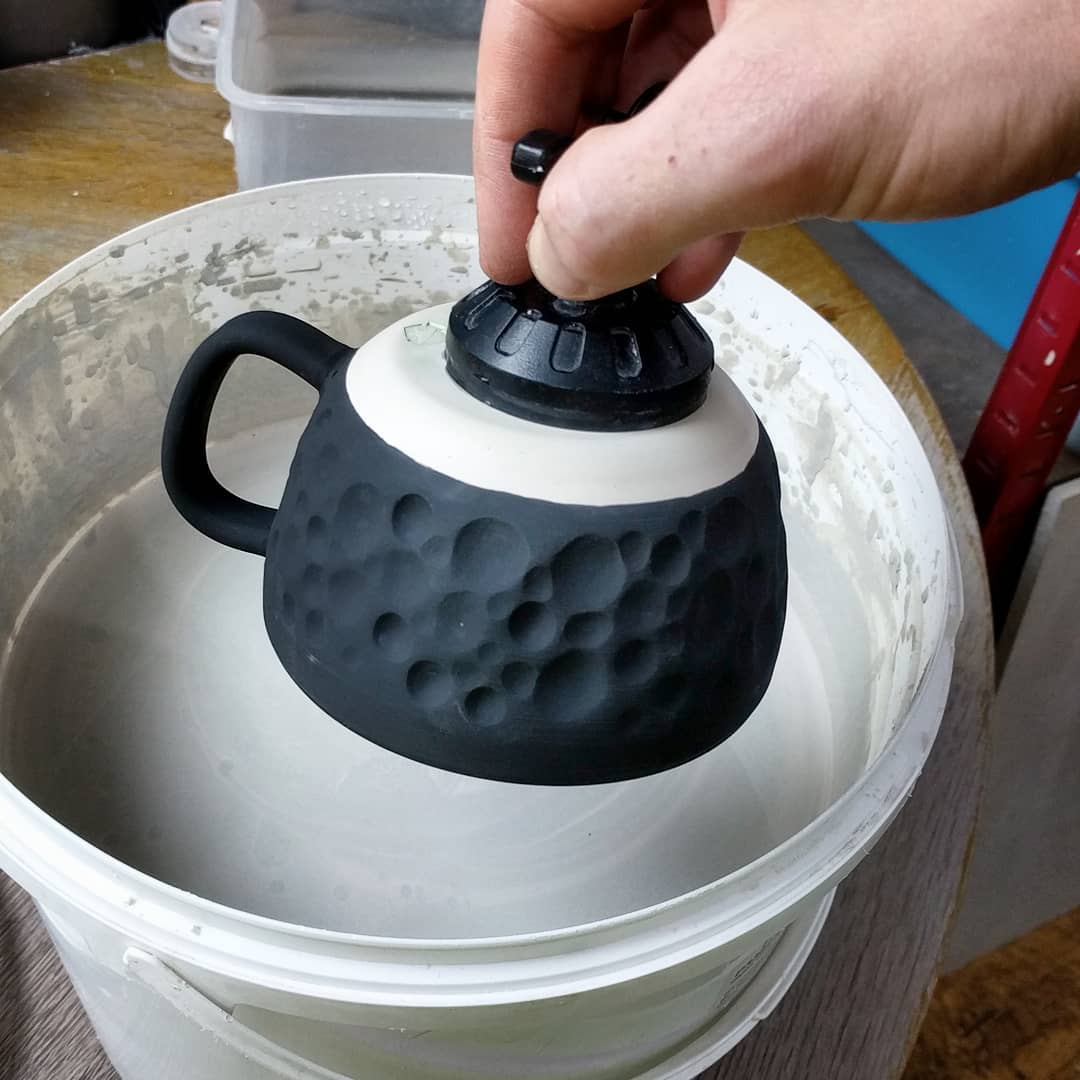In the image, a man's hand is seen holding an intricately designed ceramic object, resembling a mug with a shape akin to a teapot. The lower portion of the object is black with a cratered, moon-like texture and an overlapping pattern somewhat reminiscent of a golf ball. The craters vary in size and give it a unique, tactile surface. Towards the top, the surface becomes smooth and white. The man is grasping the object by a distinct black handle.

This ceramic piece is held upside down over a white bucket filled with a gray glaze, likely used for finishing the ceramic. The bucket itself rests on a wooden table. There's also a hint of red visible near the man's hand. The entire setup suggests a process in a ceramics class or studio, where the artist is about to dip the mug into the glaze, adding a final touch to the handcrafted piece.